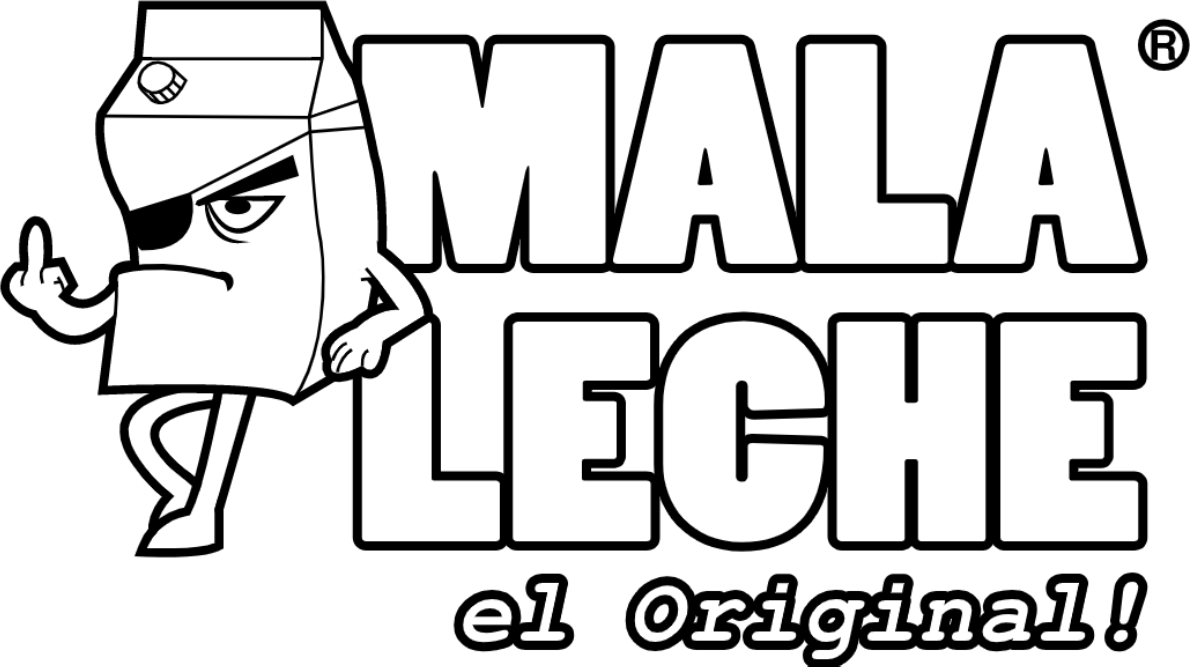The image serves as a stylized black-and-white advertisement centered around a personified milk carton, characterized by a grinning, eyepatch-wearing face. The mischievous milk carton, standing to the top left, defiantly flips off the viewer with its middle finger while leaning against the large, bold letters. The prominent text reads "Mala Leche, El Original" with "Mala Leche" displayed significantly larger to the right and "El Original" positioned in the bottom right corner. The letters and all elements are outlined in black, with the milk carton and text in white, emphasizing the stark contrast and edgy design. A registered trademark symbol (®) is located in the top right, reinforcing the brand's identity. The overall composition suggests a rebellious or non-conformist branding, highlighted by the carton character’s rude gesture and over-the-top persona.